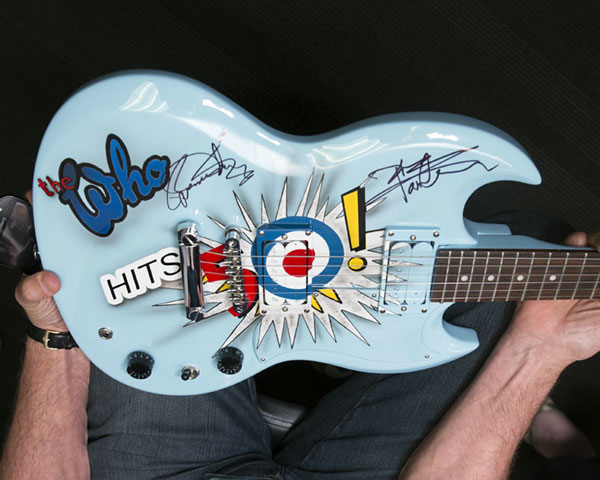This photograph captures a detailed scene of a man holding a distinctive, light blue electric guitar with a unique, curvy frame that resembles a bat wing. Only the body and part of the neck of the guitar are visible as the instrument is turned sideways and rests in the man's lap, where his hands and part of his forearms can also be seen. The guitar is adorned with multiple autographs, featuring a prominent sticker that reads "The Who" in blue. Additionally, there is a bold target symbol in the middle of the guitar, composed of blue, white, and red rings with a spiky design emanating from it, resembling an explosive burst. Another notable element on the guitar is a label that says "Hits 50," with the '0' in '50' represented as a target, encompassing red, white, and blue colors, and accompanied by a yellow exclamation point.